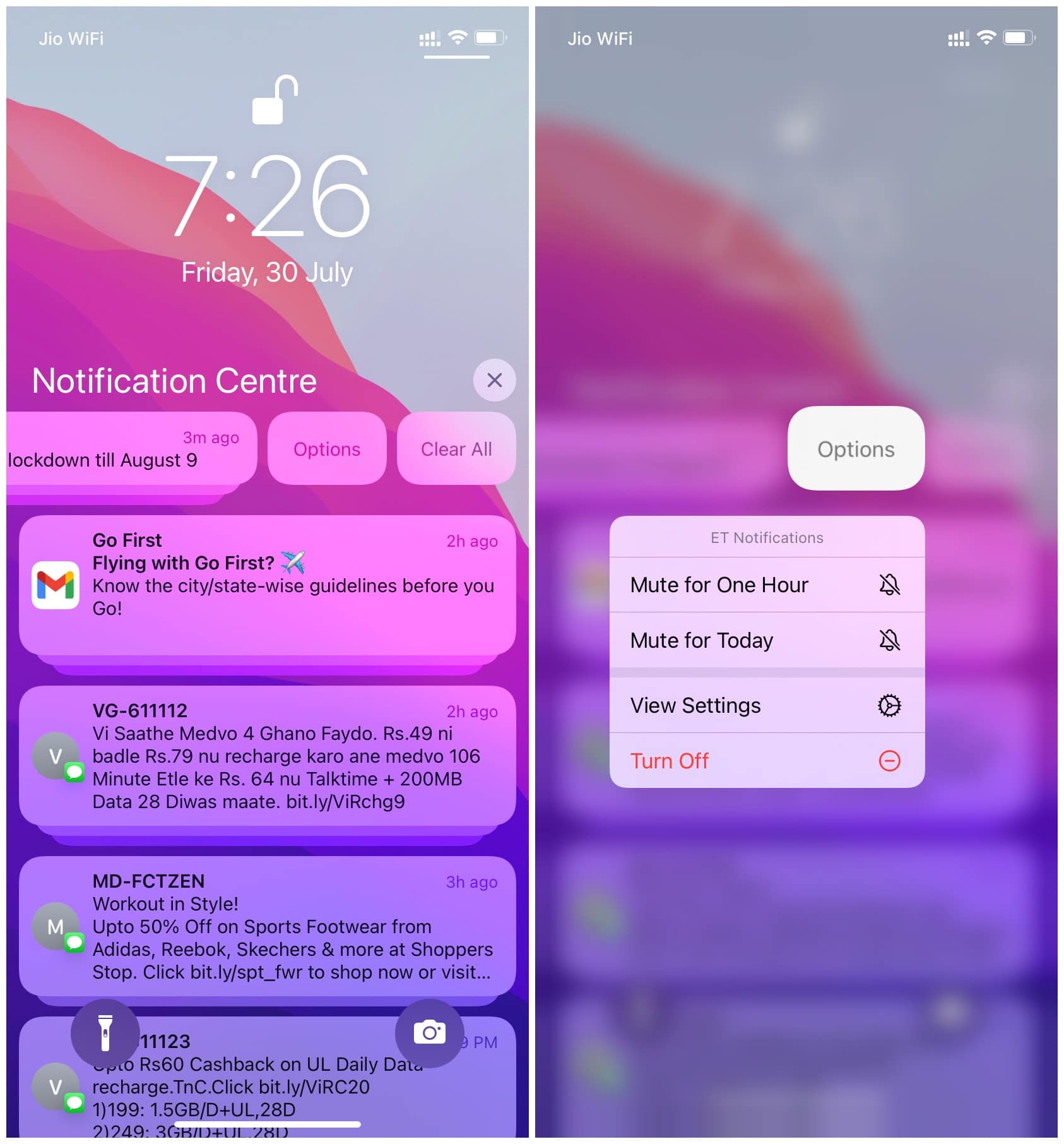This image features two mobile screenshots of lock screens placed side by side. Both screens display standard lock screen elements such as the time, date, Wi-Fi symbol, battery icon, data signal indicator, and various notifications from the notification center.

**Left Screenshot:** 
- Time displayed: 7:26
- Date: Friday, July 30
- The phone appears to be unlocked, indicated by the absence of a lock icon near the time display.
- Notifications:
  - The topmost notification has been partially swiped to the left, revealing management options like "Options" and "Clear All." The visible text reads "Lockdown till August 9."
  - Below, a multiple-stacked notification from a messaging app (indicated by a generic message icon) consists of three promotional texts, likely junk or spam mail. 
  - Furthermore, a generic notification (possibly a system alert or app notification) appears, informing the user of an update or maintenance.

**Right Screenshot:**
- The background flaunts a gradient color scheme transitioning from a purple and blue hue at the bottom to pink and orange at the top.
- The lock screen is blurred due to the selection of a notification. This blur centers around a notification management pop-up menu.
- The menu provides several options for the selected notification, including "Mute for 1 hour," "View," "Settings," and "Turn off," suggesting contextual actions for managing this specific alert.

The detailed visualization provided in these screenshots emphasizes different lock screen states and the array of notification management options available on the device.